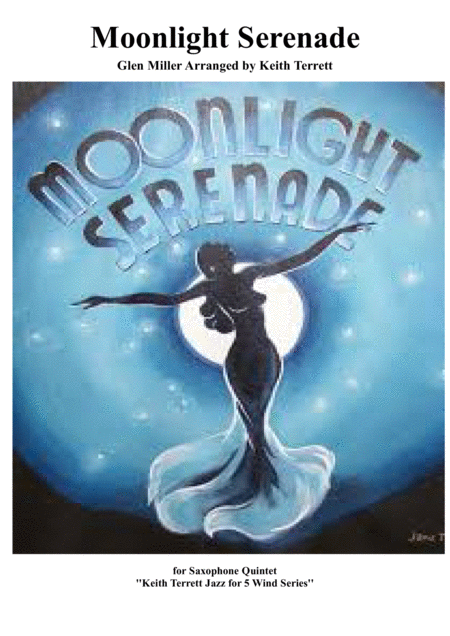The image is a highly detailed concert poster, predominantly in shades of blue and black with contrasting white elements. At the very top, "Moonlight Serenade" is written in an arc style, alternating in blue and black text. Below this, the names Glenn Miller and Keith Tarrant are mentioned, with "arranged by Keith Tarrant" specified, indicating a distinctive arrangement. The bottom of the poster features the text "for saxophone quintet" and "Keith Tarrant Jazz for Five Winds Series." 

Centrally, the poster portrays a silhouetted female figure with long, flowing hair, dressed in a mermaid-style gown. Her arms are outstretched, and she gazes upwards into a starry sky. Encircling her is a large, blue circular background filled with silver, white, and bright stars, creating a celestial ambiance. A white spotlight effect emanates from the center, highlighting the woman against the dark surroundings. The corners and ground are dominated by black, enhancing the luminous quality of the central sky and the figure's silhouette.